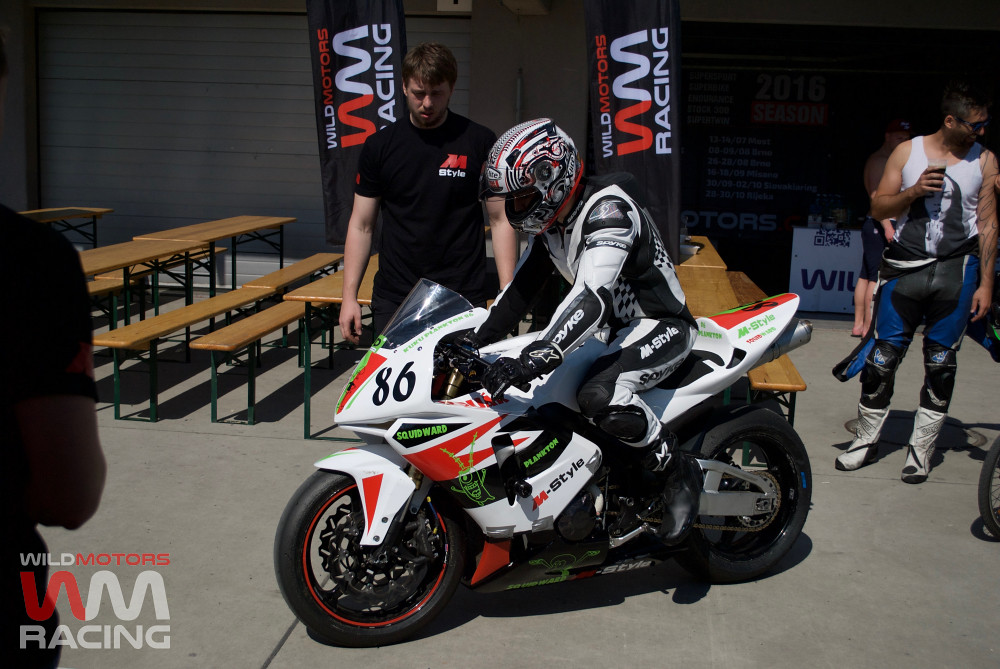This photograph captures a motorcyclist positioned directly in front of a garage surrounded by wooden benches and lunch tables. Prominently displayed above the scene are black banners featuring white and orange text that reads "WM Racing," short for Wild Motocross Racing. The rider, fully equipped in a racing suit and a multicolored helmet, is mounted on a striking white and black motorcycle adorned with various stickers, including prominent orange and black designs. The front fender bears the digits "86," while additional advertisements are visible on the side and back fenders. Notably, the motorcycle's tire is distinguished by a red stripe. To the left of the motorcyclist stands a man in a black shirt, which also features an advertisement in the upper right corner.